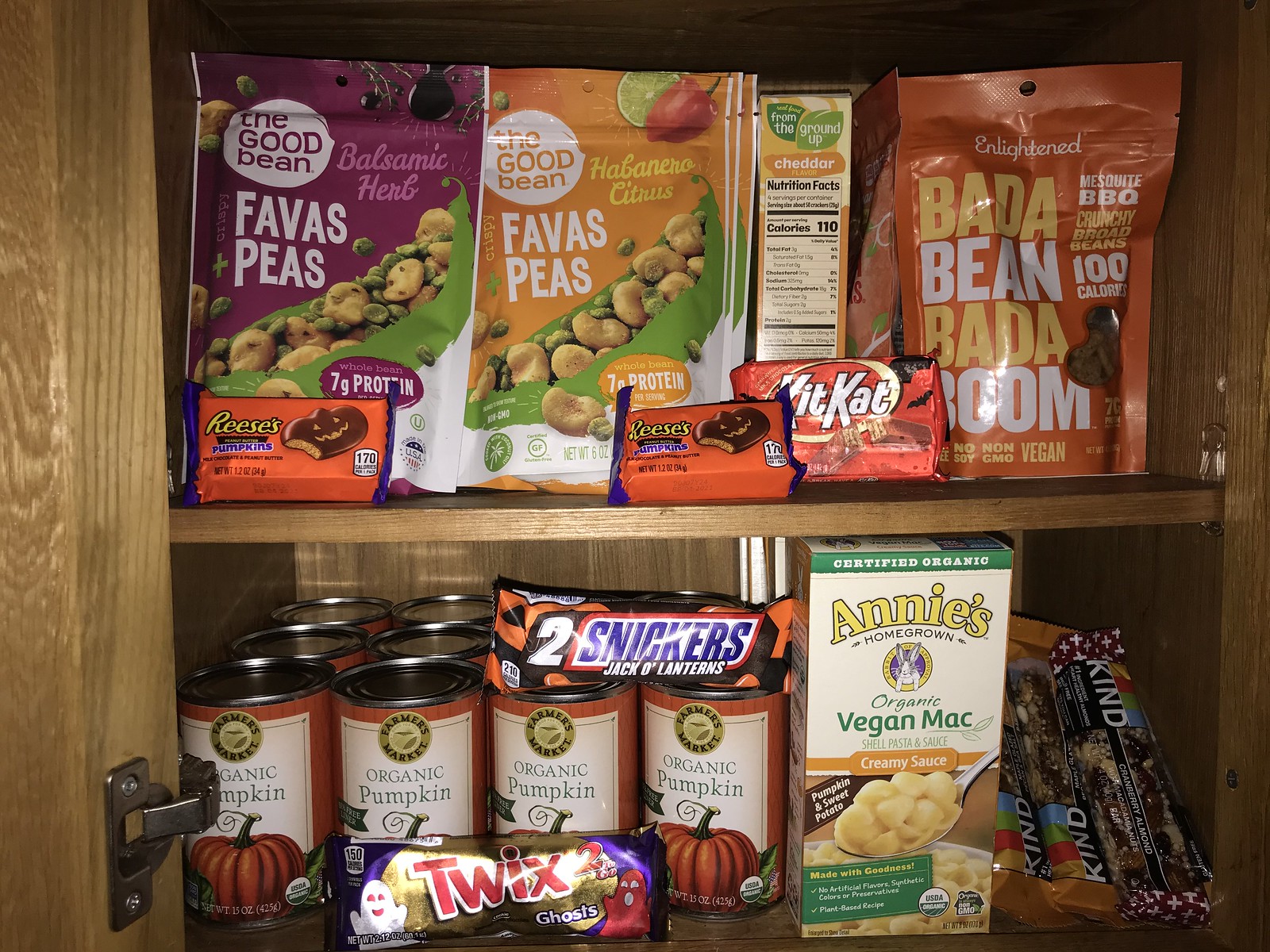This image depicts a medium-shaded brown wooden cabinet with two shelves. On the top shelf, there are several packages of snacks including a bag of fava peas with balsamic herb flavor, another bag of fava peas with habanero citrus flavor, a "Bada Bean Bada Boom" mesquite barbecue crunchy bean snack, a KitKat bar, and two Reese's pumpkins. 

In the bottom shelf, there is at least one box of Annie's Homegrown Vegan Mac, a variety of granola bars, and 12 cans labeled "Organic Pumpkin." Among the products on this shelf, there is a Snickers jack-o'-lantern positioned on top of one of the pumpkin cans, along with a package of Twix Ghosts containing two wrapped Twix bars.